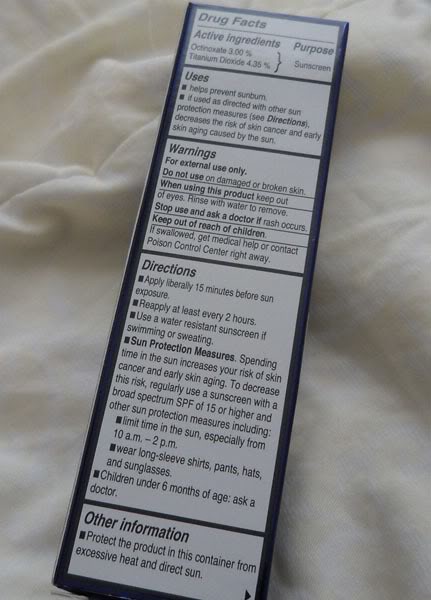This image is a close-up photograph of the back of a product box, likely for sunscreen. The box has a dark blue border and features a large, vertically oriented white label where detailed black text is presented. The background consists of a fluffy white sheet with cream-colored accents, displaying noticeable folds, creases, and shadows, especially on the top left and bottom right corners.

At the very top of the label, "Drug Facts" is prominently displayed. Below that, in various sections, the label lists important information such as "Active Ingredients," "Purpose," "Uses," "Warnings," "Directions," "Sun Protection Measures," and "Other Information." The "Uses" section mentions that the product helps prevent sunburn and, when used correctly along with other sun protection measures, can decrease the risk of skin cancer and early skin aging caused by sun exposure.

The "Warnings" section advises that the product is for external use only, should not be used on damaged or broken skin, and must be kept out of the eyes (rinse with water to remove if contact occurs). Users are instructed to stop use and consult a doctor if a rash occurs and to keep the product out of reach of children.

The "Directions" section provides guidelines on applying the product liberally 15 minutes before sun exposure and reapplying at least every two hours, especially after swimming or sweating. 

The "Sun Protection Measures" section highlights additional precautions such as limiting sun exposure between 10 AM and 2 PM and wearing protective clothing, hats, and sunglasses. It also advises consulting a doctor before using the product on children under 6 months of age.

Finally, the "Other Information" section recommends protecting the container from excessive heat and direct sun exposure to maintain the product's efficacy.